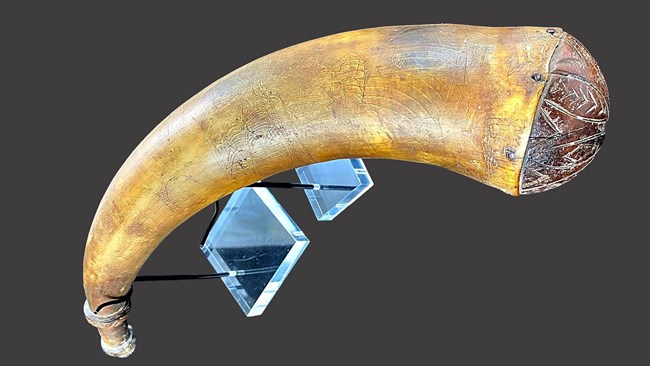This is a photograph of an antique horn or possible tusk, intricately carved with fine, hard-to-see details. The horn features a bulbous base with a circular half-circle part adorned with carvings that include, possibly, a fish with scales, and three evenly spaced nails at the base. It mounts onto two light blue diamond-shaped pieces of glass or plastic panels, one larger and one smaller, connected to the horn by a slender black wire-like structure. The horn is light brown and appears very aged, with noticeable scratches and markings suggesting it could be made of wood or some biological material. The horn narrows to a small end and curves down into a cone shape, with dark brown decorative carving at the bottom, suggesting it might have been used historically, possibly as a gunpowder container for a musket or a canteen. The overall visual suggests an old, meticulously detailed, wall-mounted artifact.